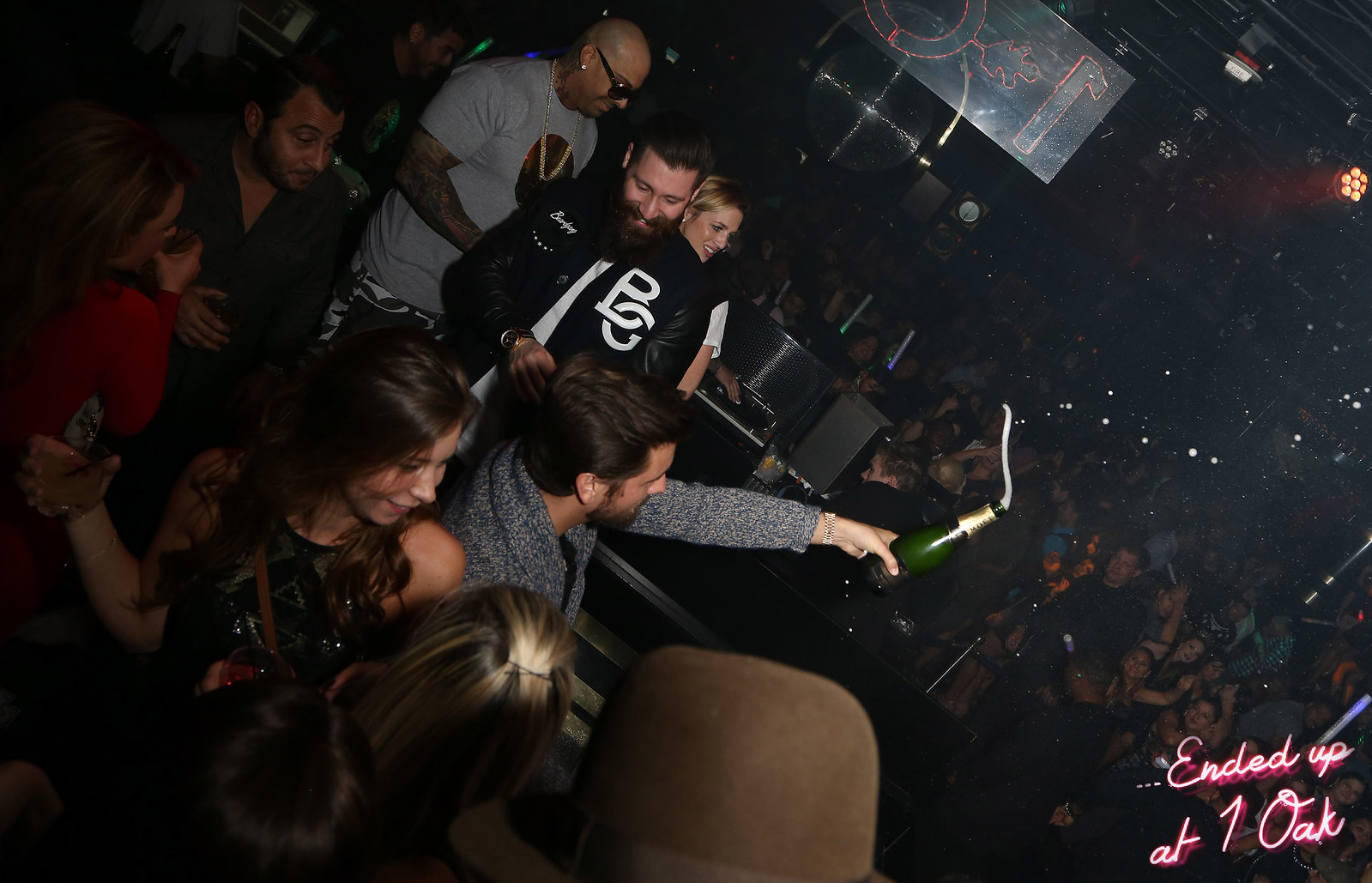The photograph captures a vibrant nighttime scene at a crowded nightclub, likely One Oak, as indicated by the neon pink text in the lower right corner. The setting is dark with minimal lighting, emphasizing the party atmosphere. The image seems to be taken near the DJ booth, slightly elevated above the dense crowd. Central to the image is a man with dark hair and a beard wearing a gray long-sleeved shirt, holding a champagne bottle from which a stream of champagne is seen shooting out. To his side, a woman with dark hair engages in conversation with another woman whose blondish hair is visible from the back. In the background, additional figures can be seen, including a man in a black jacket with white lettering, another man in a gray t-shirt with sunglasses, and a few other partygoers dressed for a night out. The crowd below adds to the lively scene, with dancing and celebration taking place under the nightclub's ceiling lights.